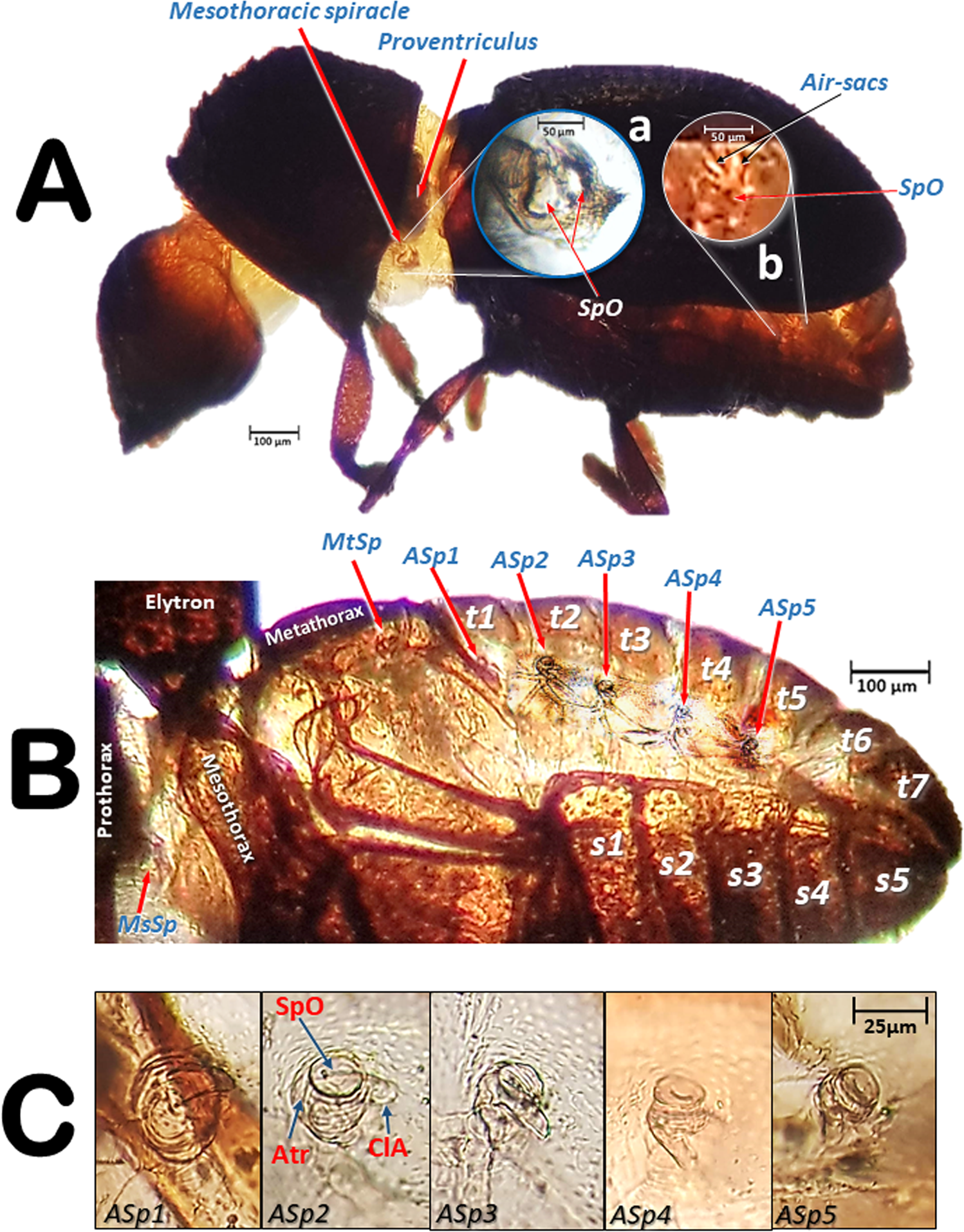This detailed scientific diagram showcases the anatomy of a bee, intricately labeled with various sections of its body, and includes enlarged views for detailed examination. The diagram features three main images labeled A, B, and C. Image A displays the overall structure of the bee with numbered labels indicating different anatomical parts such as the proventriculus and mesothorax spherule. Image B zooms in on the bee's stinger, highlighting its specific components. Image C provides a microscopic view, featuring five detailed images that further explore the intricate structures of the bee's anatomy. The consistent amber color unifies the series, making it a comprehensive and educational piece, suitable for a biology textbook.